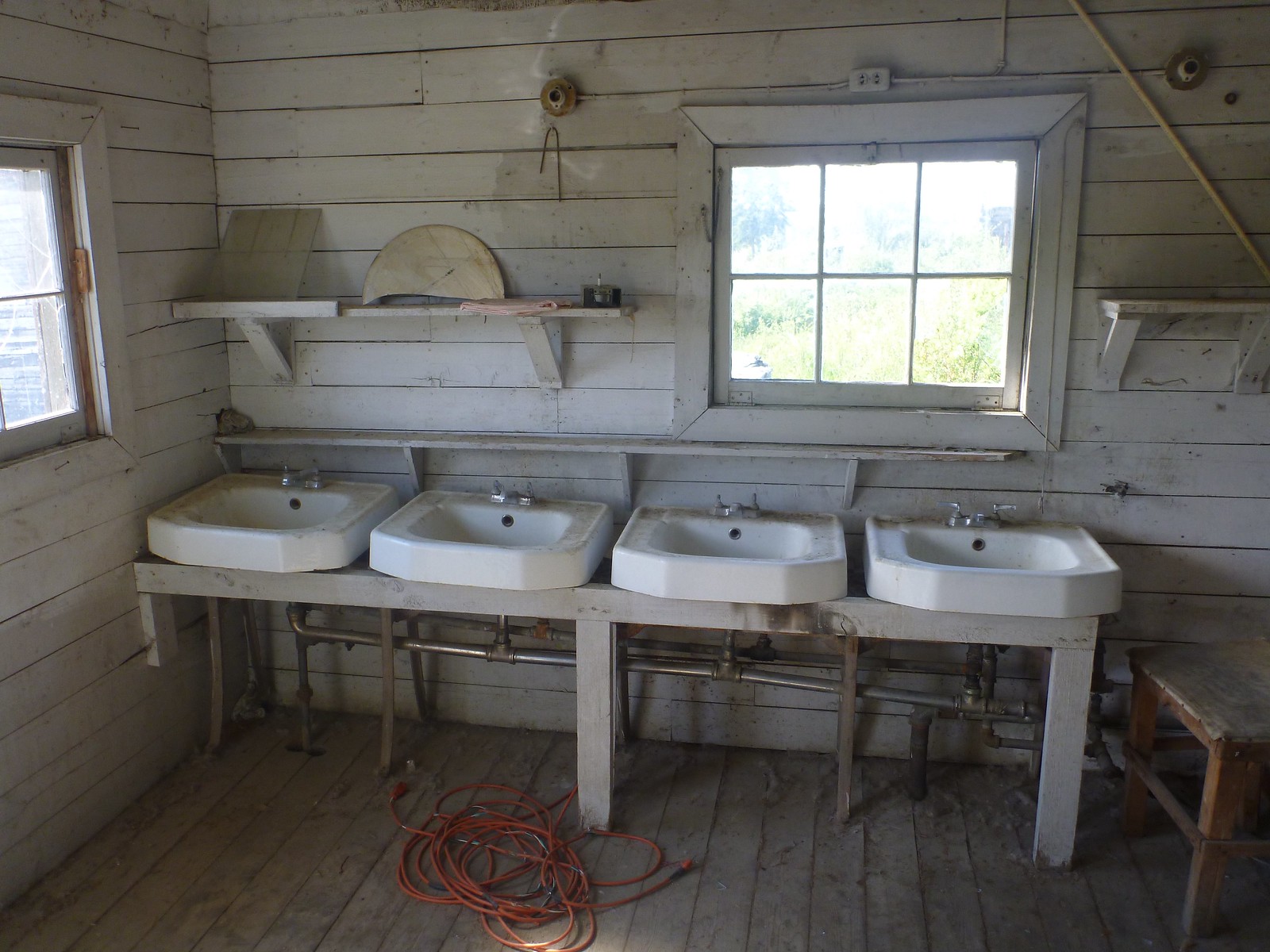The image depicts the interior of an old, rustic bathroom within a barn or shed. The walls are made of horizontally slatted, whitewashed wooden panels that exhibit signs of aging. The focal point of the room is a row of four white, rectangular porcelain sinks, each equipped with metal faucets and underpinned by white legs. The sinks are mounted on a single wooden beam with visible plumbing running beneath them, connecting all the sinks together. Above the sinks, there are small white shelves, holding miscellaneous objects, while higher up, wider shelves accommodate several items.

The room features two panelled windows: one on the left wall and another directly in the middle, both framed in white. These windows are divided into six small panes each, allowing sunlight to filter through and illuminate the space. The floor is composed of wooden planks, on which rests a coiled orange extension cord in front of the sinks. To the right of the sinks, there is a small wooden table, contributing to the rustic ambiance of the room. The overall appearance of the interior suggests a utilitarian setup, with an emphasis on functionality over aesthetics, reflecting the room's age and wear.